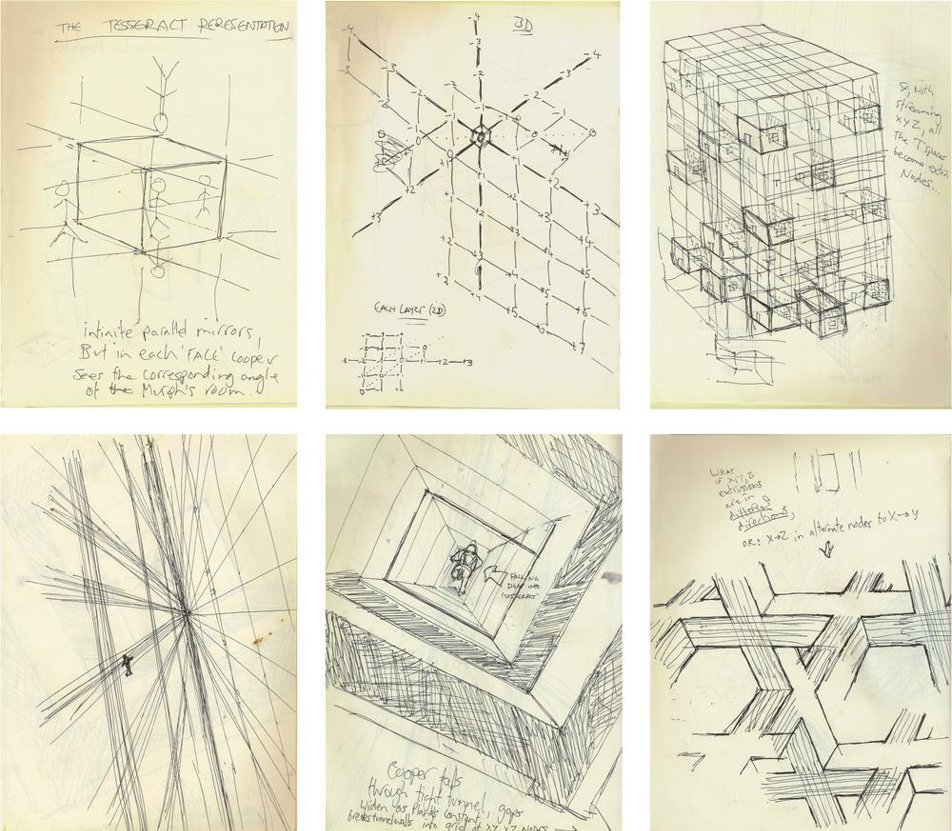The image consists of six detailed pencil or ink sketches arranged in a 3x2 grid on yellow paper. Each drawing is on a separate rectangular sheet with spaces in between, creating a cohesive collage. The top-left sketch illustrates a cube with at least one stick figure inside and two observing from the outside, with an inverted figure above. It is titled "The Tesseract Presentation," with a caption beneath reading, "Infinite parallel mirrors but in each face Cooper sees the corresponding angle of Murph's room." Adjacent to it on the top row, the second sketch features numbered cubes and squares, configured to appear three-dimensional. The third image depicts a large, complex array of cubes blending into each other. The bottom-left drawing presents a grid-like structure, while the bottom-center sketch illustrates a figure running through a maze-like tunnel filled with cubes, annotated with "Cooper falls through tight tunnel, gaps widen as planes constant, breaks tunnel walls into grid." The final sketch at the bottom-right showcases a maze with textual elements at the top, drawn in either pen or pencil.